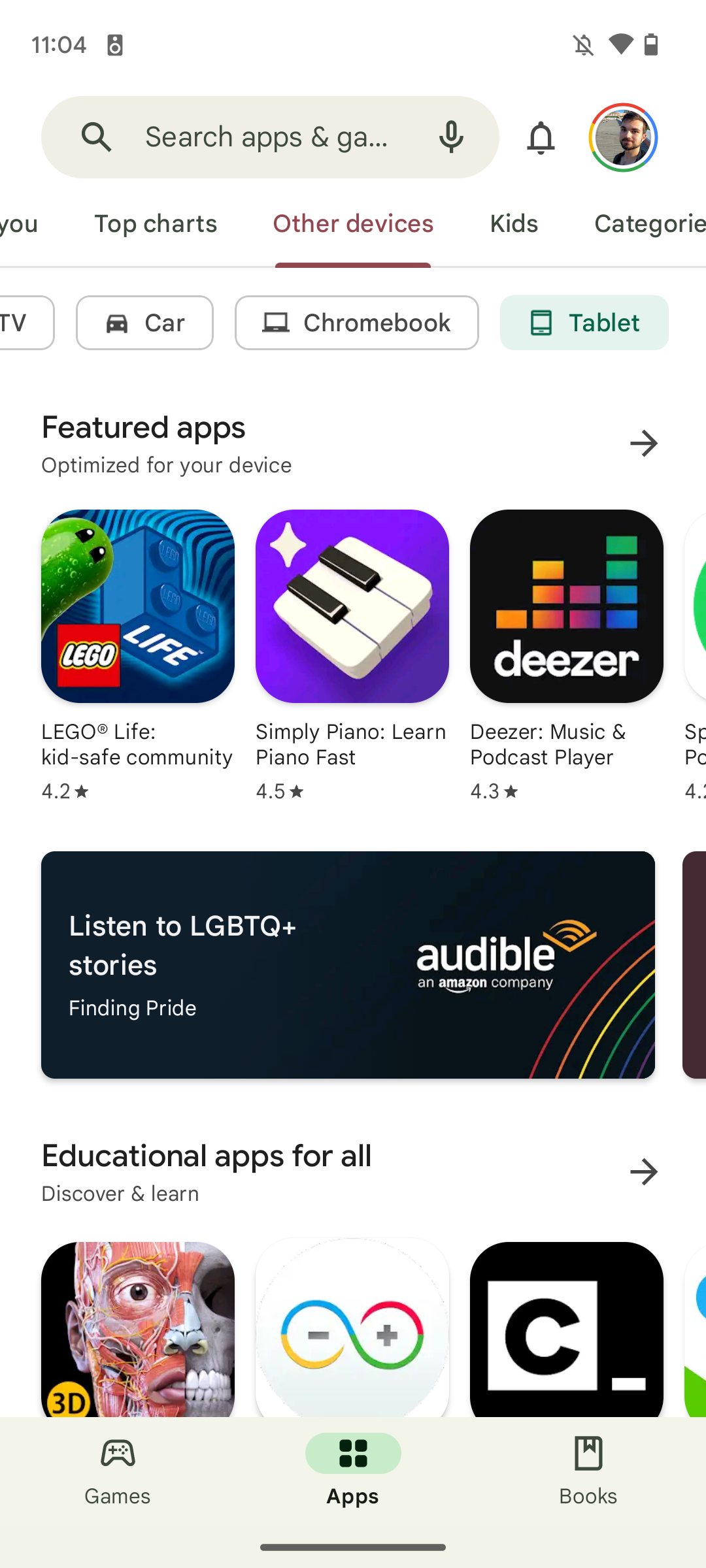The image is a screenshot taken from a smartphone, showcasing a section of an app store interface. The background of the interface is predominantly white. At the very top of the screen, the time is displayed as 11:04, with the battery icon indicating it is about halfway charged. The Wi-Fi icon shows that the device is connected to a network, and notifications are turned off.

Underneath the status bar, there is a man's profile picture located on the right side of the screen. Adjacent to the profile picture, in the center, there is a bell icon. On the left side, there is a search bar labeled "Search apps and games."

Below this header, a navigation menu is visible with tabs including "Top charts" and "Other devices," with "Other devices" being highlighted in red. Additional tabs such as "Kids," "Categories," "Car," "Chromebook," and "Tablet" are also present.

As you scroll down, you encounter a section titled "Featured apps," which offers a selection of optimized apps for the device. Visible apps in this section include "LEGO Life," "Simply Piano: Learn Piano Fast," and "Deezer: Music & Podcast Player." Some app titles are partially cut off from the screenshot.

Further down, another section titled "Listen to LGBTQ+ stories: Finding Pride" from Audible is displayed. Additionally, there's a mention of "Educational apps for all," suggesting another category of available applications.